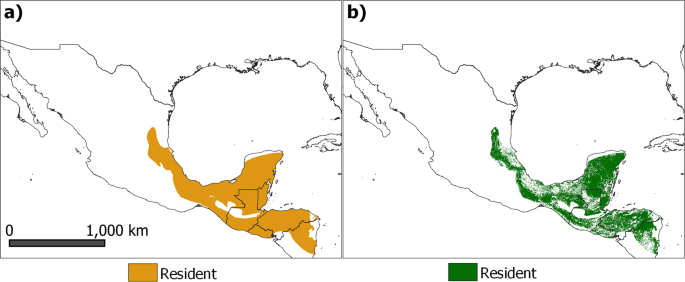The image features two side-by-side, square, black-outlined maps of Mexico with minimalistic designs against a white background. Both maps are labeled boldly in the upper left corners: the left map as "a)" and the right map as "b)". In the lower left corner of the left map, a black bar indicates a scale from 0 to 1,000 kilometers.

Map "a)" highlights portions of the southern region of Mexico in a dark mustard color, corresponding to a rectangle below the map labeled "resident" in the same dark mustard shade. Adjacent to it, map "b)" highlights identical regions but in dark green, paired with a coordinating green rectangle below, also labeled "resident". The outlines of both maps are simple, black sketches, delineating the geographic boundaries of the highlighted regions.